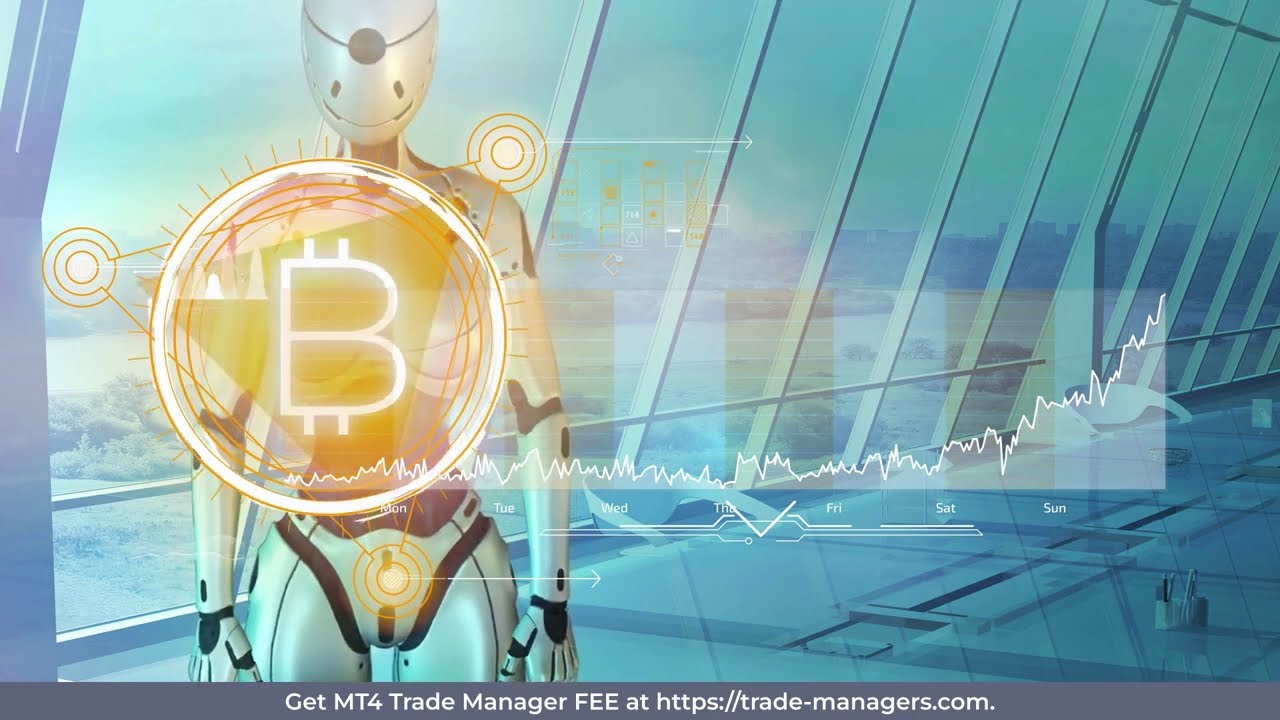The image depicts a technologically advanced and futuristic scene set in a large building with expansive, glass-paneled windows, through which a hazy cityscape can be seen. Dominating the left side is a sleek, silver robot with a human-like form, featuring a white and black armored body. The robot's head sports a black headband and black eyes with a small smile, and its joints have black accents. In the forefront of the image, a prominent Bitcoin symbol— a 'B' with two horizontal lines at the top and bottom— is enclosed within a circle and interwoven with a triangular graphical figure. Along each point of the triangle, there are sets of concentric circles adding to the high-tech aesthetic. Anchoring the composition, a line graph is displayed in the background, charting data from Monday to Sunday, showing a gradual rise before a sharp increase on Sunday. The image is overlaid with a promotion, in white text within a gray rectangle at the very bottom, stating, "Get MT4 Trade Manager Fee at https://trade-managers.com."